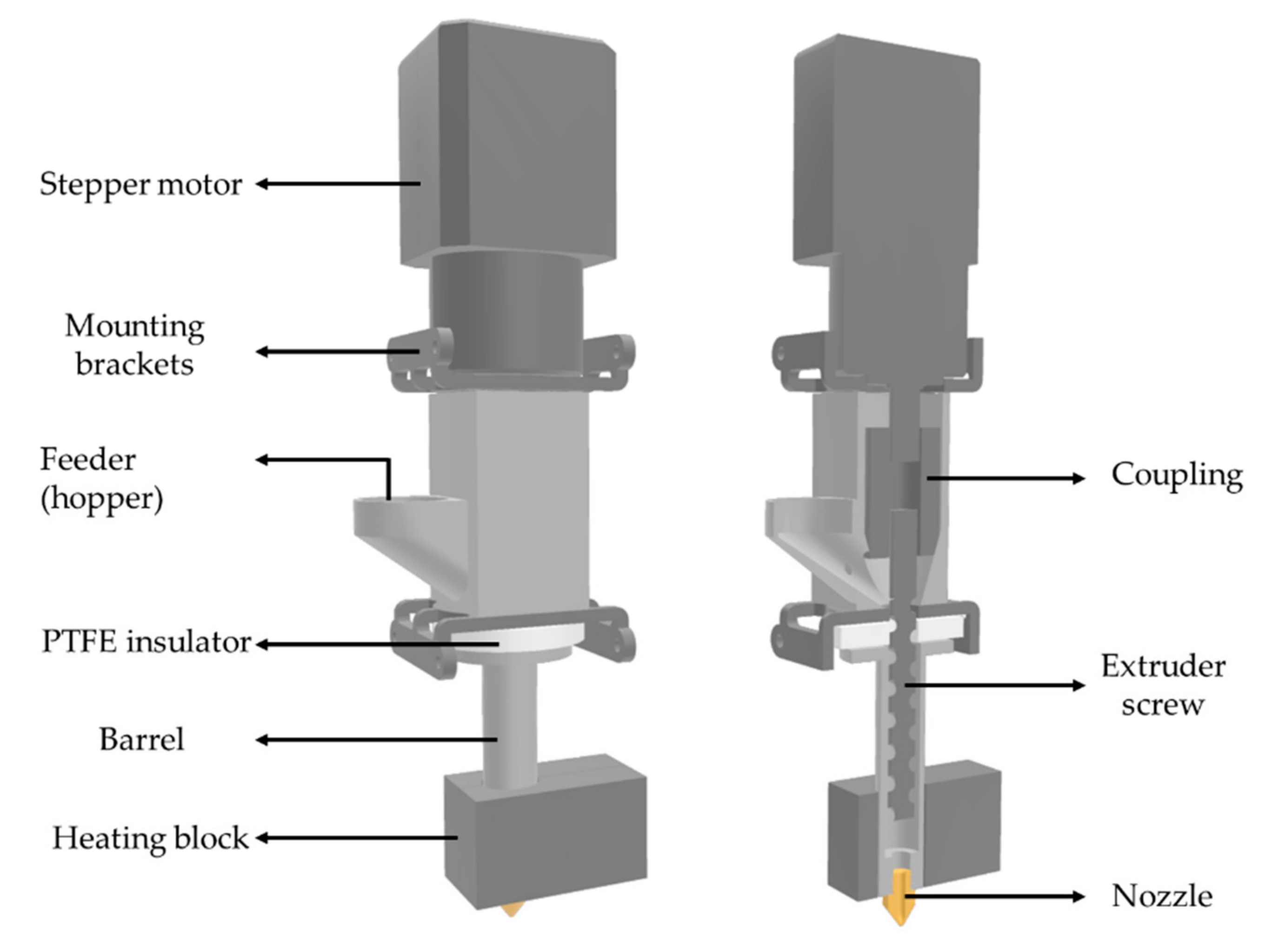This image features a detailed 3D rendering of the printing head of a 3D printer, depicted in various shades of gray. The rendering is shown from two perspectives: an exterior view on the left and a cross-sectional view on the right. The composition appears on a white background with no definitive borders. Key components are labeled with black text and arrows. 

Starting from the top left, the labels identify a stepper motor, followed by mounting brackets, a feeder (or hopper), a PTFE insulator, a barrel, and a heating block. In the cross-sectional view on the right, labeled components include a coupling, an extruder screw, and a nozzle. Notably, the nozzle stands out in a yellowish-gold color. 

The overall design lacks physical markings and appears to be a digital illustration, possibly created for instructional purposes such as a manual or CAD documentation. The detailed labeling and cutaway view help clarify the internal structure and function of the 3D printer head, resembling the compact, vertically-oriented configuration of a motor-driven extrusion system.